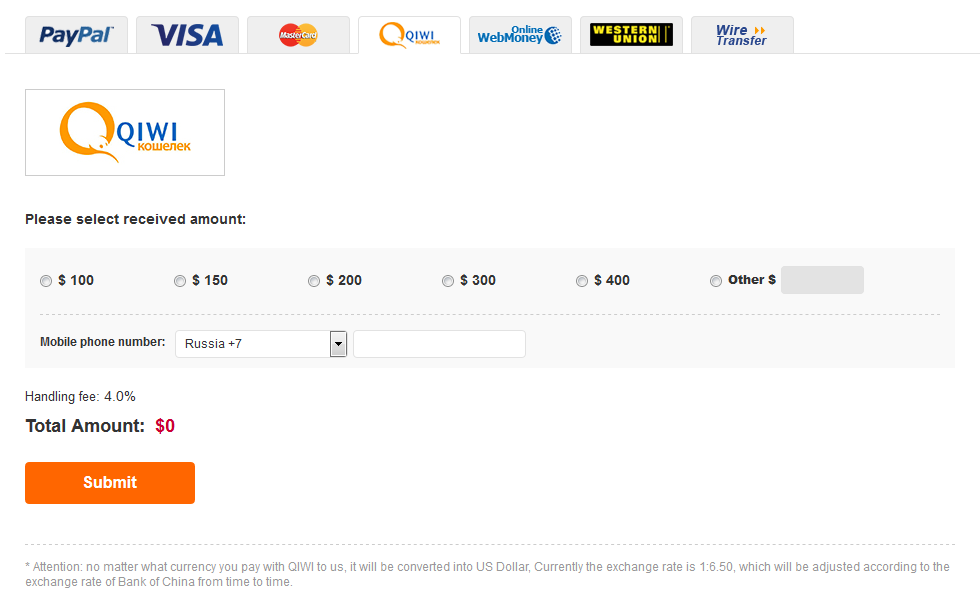A detailed screenshot of a payment selection and processing page displaying options and instructions for completing a transaction. The interface includes a dropdown menu labeled "Please select received amount" with multiple options: 100, 150, 200, 300, and 400, as well as an "Other" option for custom amounts. There is a field for entering the mobile phone number and a selection labeled "Russia" indicating the processing country. Additional information includes a handling fee calculated at 4%, a total amount initially shown as zero, and a "Submit" button for finalizing the transaction. The payment methods accepted are prominently listed: Kiwi, PayPal, Visa, MasterCard, WebMoney, Western Union, and wire transfer. Each of these payment methods is repeated multiple times throughout the text, emphasizing their availability.